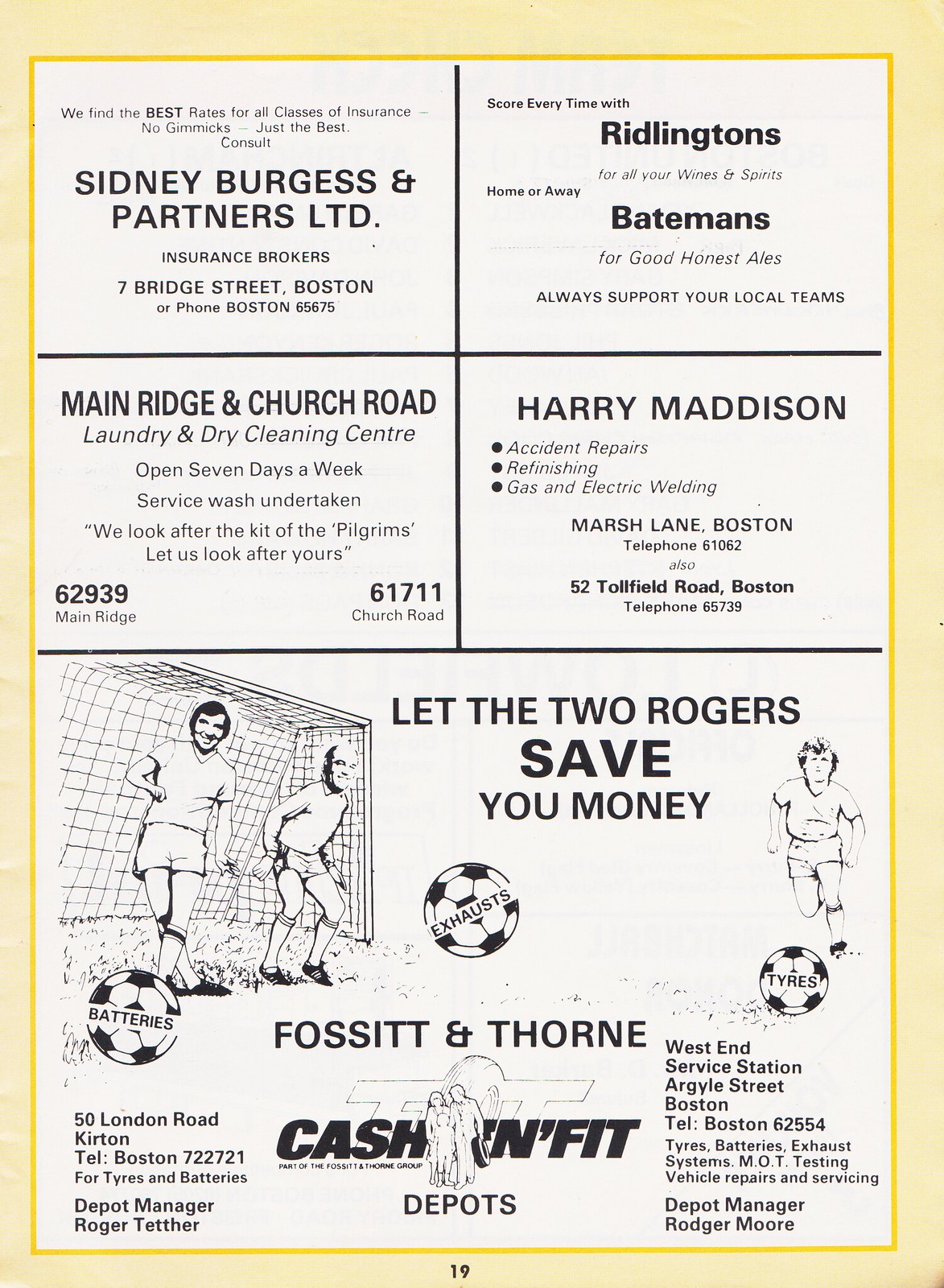This image appears to be a poster or program page with a light tan border and a thin yellow inner border, segmented into four identical rectangles at the top and one large square at the bottom. The top left rectangle features an advertisement for Sidney Burgess and Partners Limited Insurance Brokers, offering competitive rates for all insurance classes without gimmicks, and providing contact details at 7 Bridge Street, Boston, and phone number Boston 65675. Adjacent to this, the top right rectangle advertises Riddlington's for wines and spirits, and Bateman's for ales, with a message to support local teams. The bottom left rectangle promotes Main Ridge and Church Road Laundry and Dry Cleaning Center, open all week and responsible for cleaning local soccer team kits, with contact numbers 62939 for Main Ridge and 61711 for Church Road. The bottom right rectangle is an ad for Harry Madison's accident repair services, which includes refinishing and gas and electric welding, listing two locations: Marshall Lane (phone 61062) and 52 Tullfield Road (phone 65739) in Boston. The large square at the bottom showcases an illustration with a soccer goal and players, where the message "let the two Rogers save you money" is prominently displayed. On the left side, Fawcett and Thorne is mentioned, with contact details for the Cash and Fit Depots at 50 London Road, Curtin (phone Boston 722721), managed by Roger Tether, and Weston Service Station, Argyle Street, Boston (phone Boston 62554), managed by Roger Moore, offering a range of automotive services including tires, batteries, exhaust systems, MOT testing, and vehicle repairs.